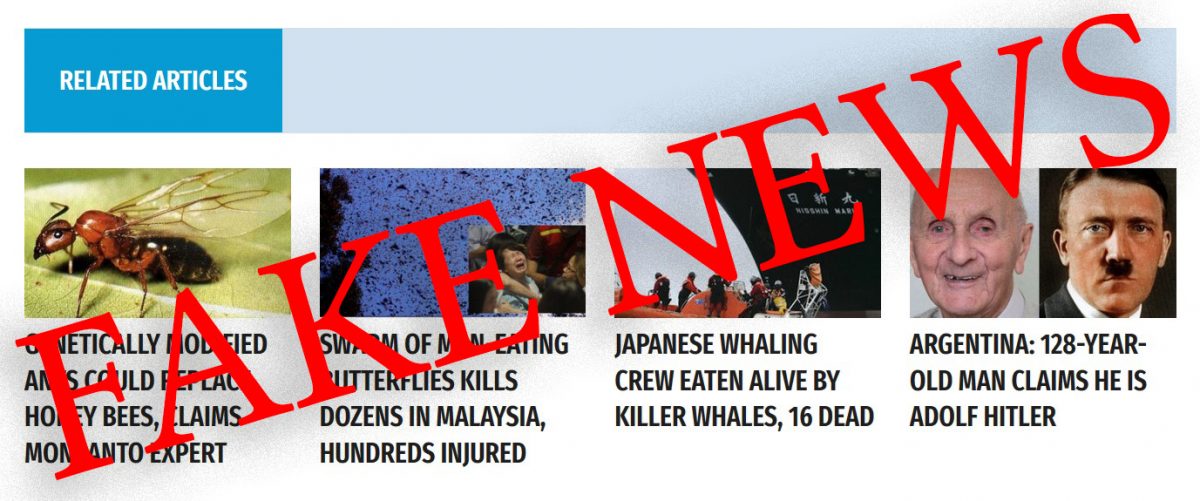The image captures a screen of a webpage displaying news articles. The webpage is structured with four smaller, side-by-side images at the center, each accompanied by a headline beneath it written in black text. Dominating the top section of the image is a blue horizontal bar featuring the phrase "Related Articles" in white text positioned to the left, on a darker blue segment of the bar. Strikingly, across the entire image at a diagonal angle, large bold red text declares "Fake News."

Adding a unique element to the image, below the four smaller images with news headlines, is the image of a brown ant. The ant is perched on a pale olive green leaf, appearing distinctly to the left side of the smaller images. The composition suggests a critique or alert about the authenticity of the news articles presented.